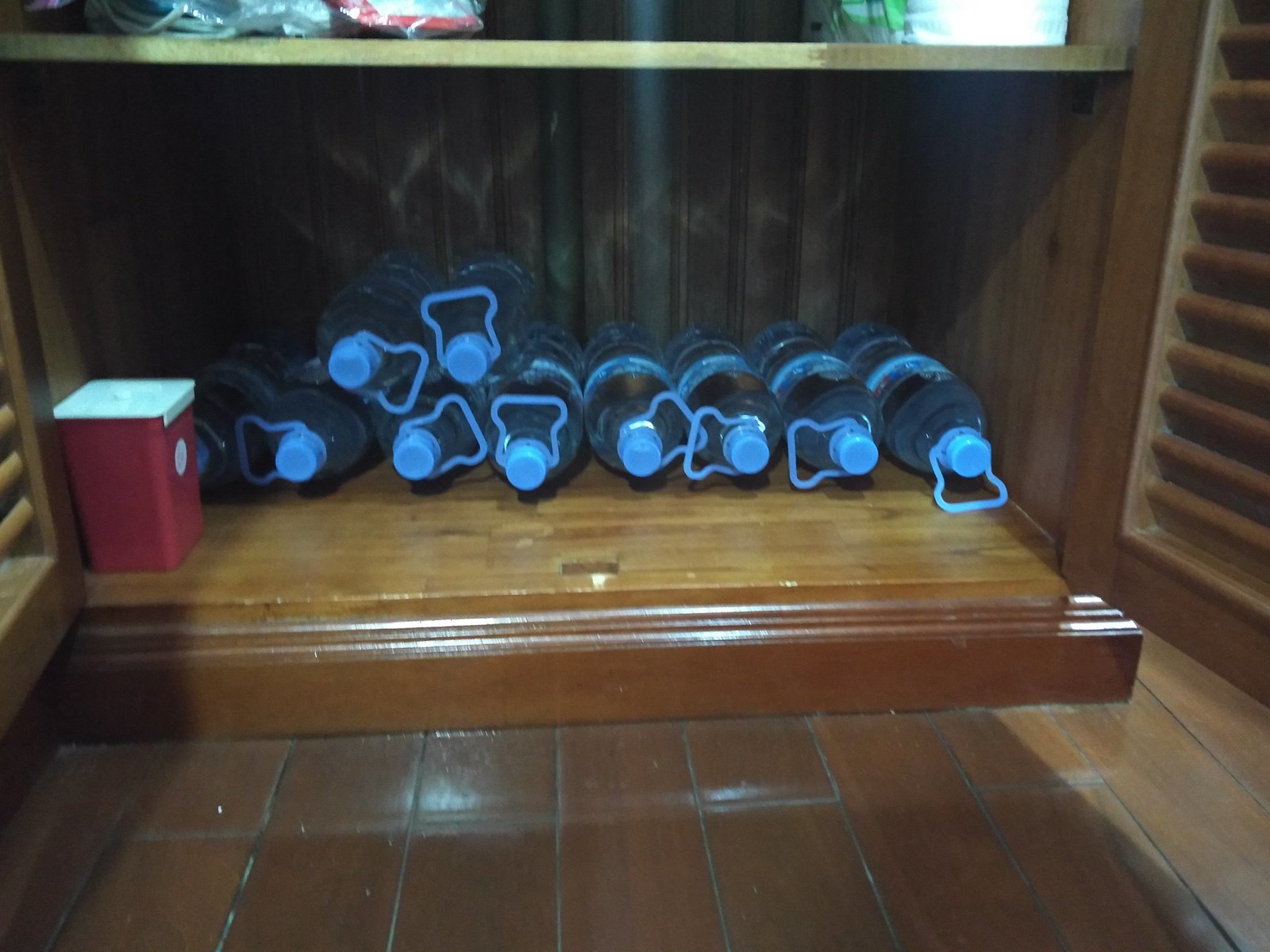This indoor photograph captures a storage area with a wooden brown floor and a matching wooden cupboard or closet. Situated on the bottom shelf of this cupboard lies an array of 10 large water bottles, each at least a gallon in size. These bottles, made of clear plastic, feature baby blue caps and handles, and are neatly positioned on their sides with the caps facing outward. Adjacent to the bottles, on the left side, there's a small red container with a white lid, resembling a medical waste disposal bin. Above the shelf holding the water bottles, another shelf is partially visible, but the items on it are not clearly discernible. The cupboard doors are shuttered and open, revealing the organized contents against a backdrop of deep brown hardwood flooring.